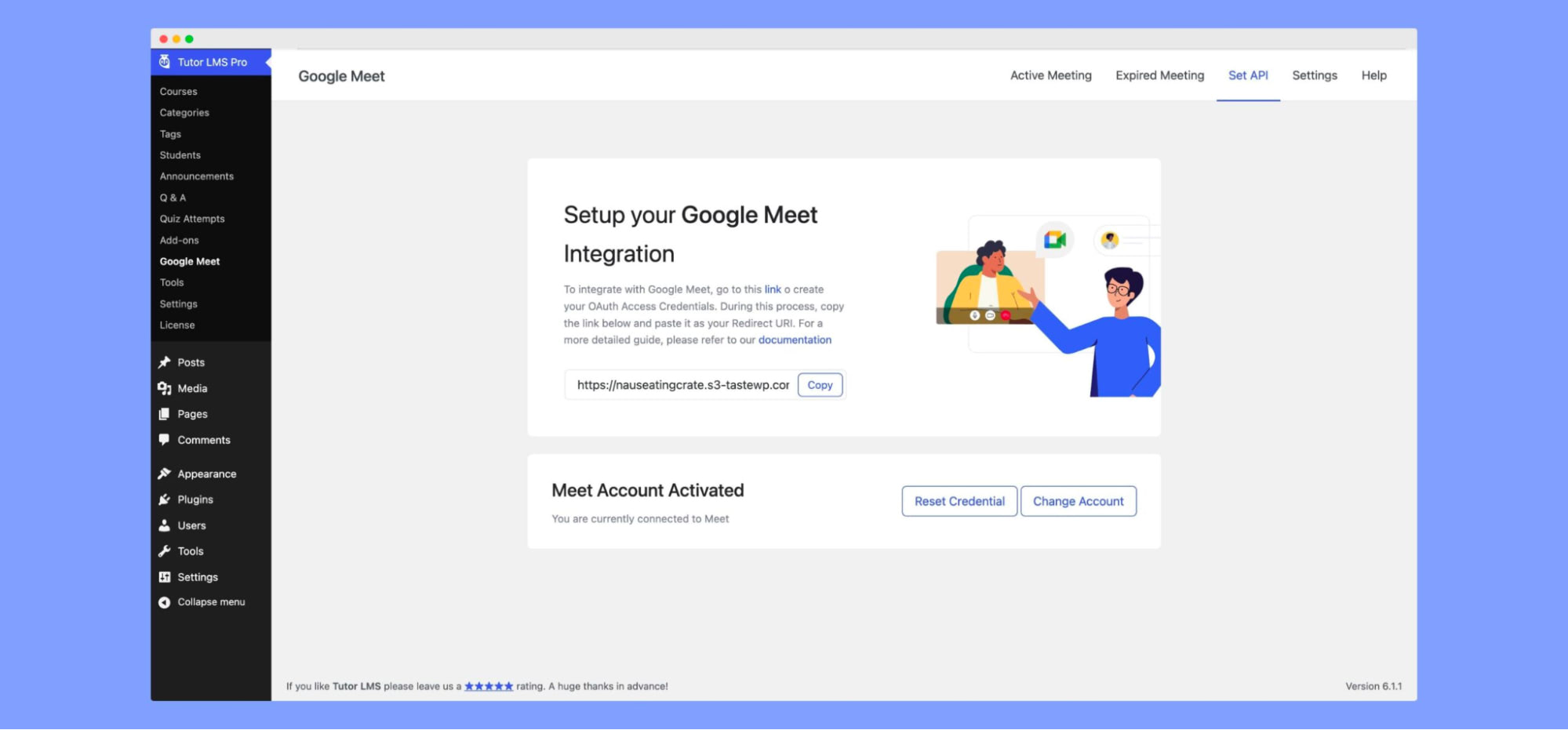This image is a screenshot of a Google Meet interface. In the upper left-hand corner, the text "Google Meet" is prominently displayed. On the upper right-hand corner, there are several menu options listed: "Active Meeting," "Expired Meeting," "Set API Settings," and "Help." The "Set API" option is highlighted with blue text and a blue underline, indicating it is currently selected. 

The center of the screen features the heading "Set Up Your Google Meet Integration," accompanied by some explanatory text and a link that users can copy. Beneath this section, a status message reads "Meet Account Activated. You are currently connected to Meet." Two actionable buttons labeled "Reset Credential" and "Change Account" are available for user interaction.

Additionally, there is a small illustration depicting one person showing another person on a screen in a virtual meeting. On the far left side of the page, there is a vertical menu with several options displayed in white text against a black background. The menu header reads "Tutor LMS Pro," although the specific menu options are hard to discern due to their small font size.